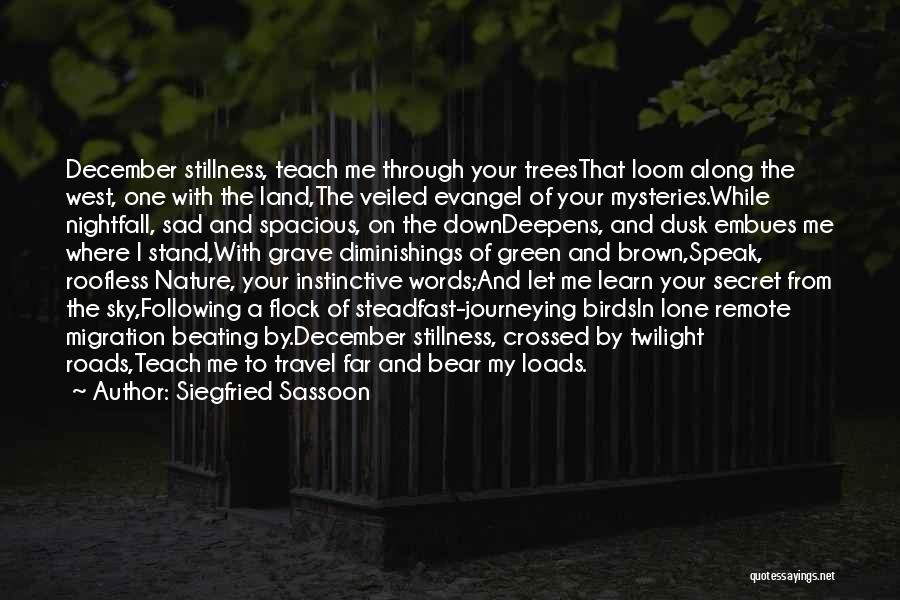This image features a dark background with a superimposed quote in bold white text that stands out prominently. The scene appears to be set in a park, with visible trees and a small structure, suggesting an outdoor setting. The detailed background includes a potted plant with green leaves, enhancing the natural ambiance of the image. Positioned prominently in the center, the quote reads:

"December stillness, teach me through your trees that loom along the West, one with the land, the veiled evangel of your mysteries. While nightfall, sad and spacious, on the down deepens, and dusk imbues me where I stand, with grave diminishings of green and brown, speak, roofless, nature, your instinctive words, and let me lean, learn, that is, let me learn your secret from the sky, following a flock of steadfast journeying birds, in lone remote migration, beating by. December stillness, crossed by twilight roads, teach me to travel far and bear my loads."
 
The quote is attributed to Siegfried Sassoon, with a subtle mention of its source, Quotesayings.net, in small text at the bottom right corner.